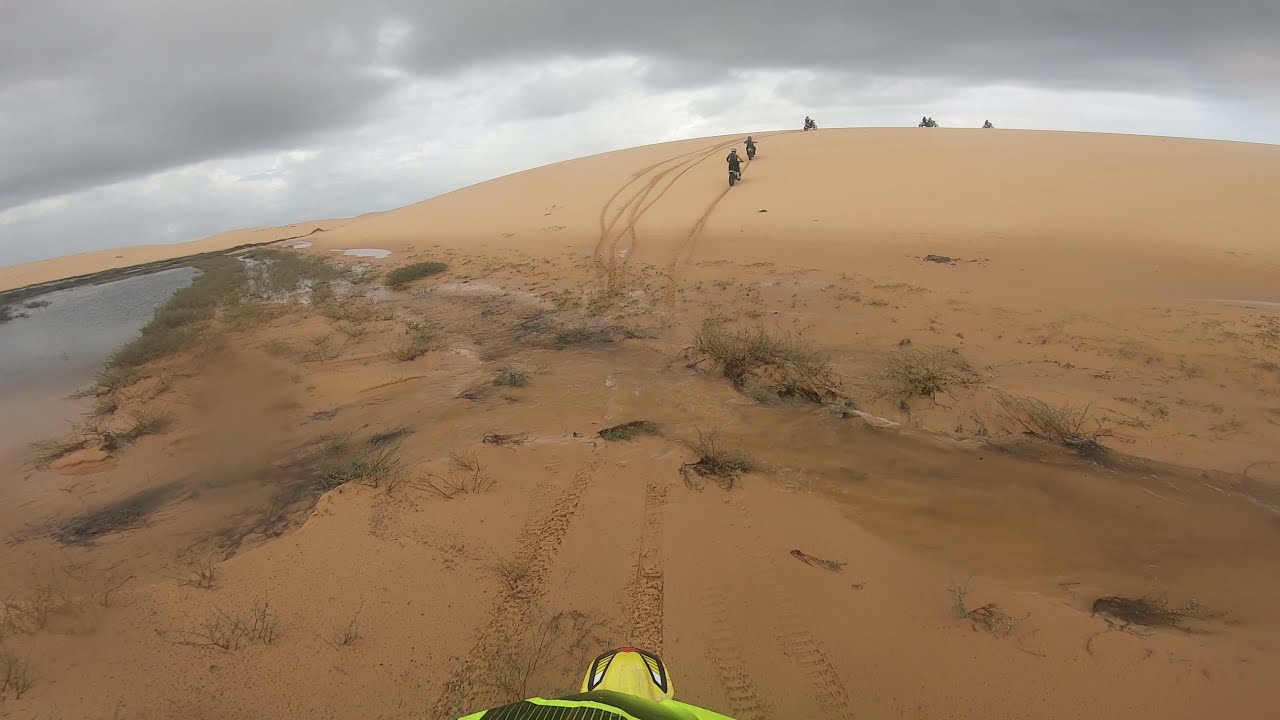The photo shows a dynamic scene from the point of view of a dirt biker navigating through sandy trails. The landscape is primarily composed of expansive dirt roads and sand dunes with numerous tracks zigzagging in all directions. On the left side, there is a small body of water, possibly a pond rather than a lake, suggesting recent rainfall. In the distance, five to six other dirt bikers, all dressed in black, are riding up a hill, with their individual paths snaking and branching out. The dirt bike in the foreground has yellow and green parts - with the wheel cover being yellow and the handle area green. The entire area is devoid of any buildings or cars, emphasizing the remote, rugged terrain tailored for off-road adventures.